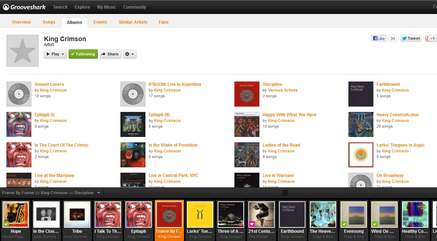The top section of the image presents a detailed overview of a music application interface. It includes a group chart that allows users to search and explore various musical elements such as songs, albums, events, and artists. The interface further features sections dedicated to artist content, playlists, and fan interactions. Users can access their music through their phones and share their favorite tracks and albums with ease.

The display showcases album covers prominently, and there is an intriguing element where album covers might feature expressive imagery, possibly depicting emotions like screaming. Users are given the option to rate or share albums directly from this interface.

The visual design is highlighted by a palette of colors including a purple icon, a green checkmark, a mix of white, red, yellow squares, and several pink and green elements, each marked with a checkmark. Text elements are also present within the interface, ensuring users can easily navigate through the different features and options available.